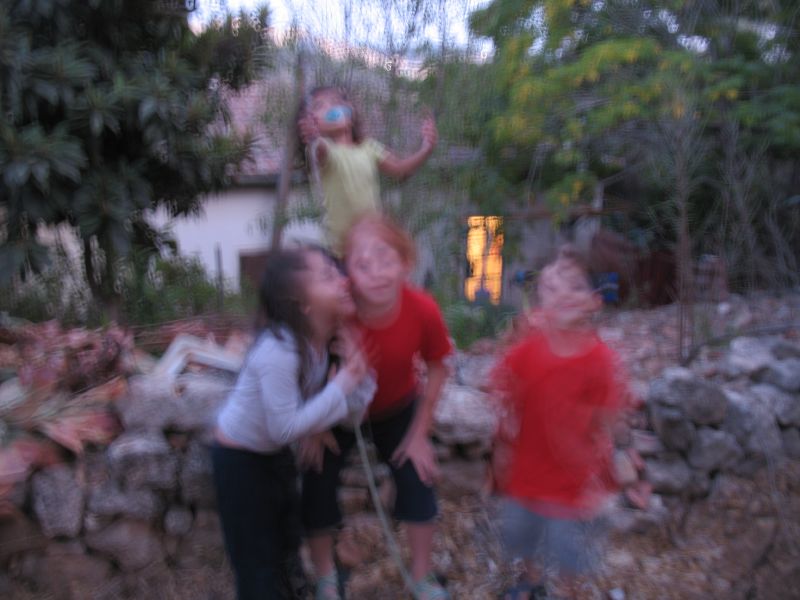This is a very blurry color photo taken outdoors in what looks like a backyard. The image, which is out of focus, showcases four children with indistinct facial features. Three children are posing in the front, backed by a stone rock wall, while the fourth child stands elevated on the wall behind them. 

The child on the left, with dark hair, is side-profiled to the right, wearing a long-sleeve white shirt and black pants, and appears to be Caucasian. Next to them is a red-haired child facing the camera. This child, also Caucasian, is wearing a short-sleeve red shirt, denim cropped pants, and white shoes, and is leaning forward with both hands on their thighs. 

Beside the redhead, there is another child who is very blurred, with dark hair styled in two ponytails. This child is wearing a red shirt and denim shorts. 

Behind them, standing on the stone wall, is a younger child with dark hair, wearing a yellow shirt and holding something that might be a blue pacifier. 

In the background, there is a house with a window that has its light on.